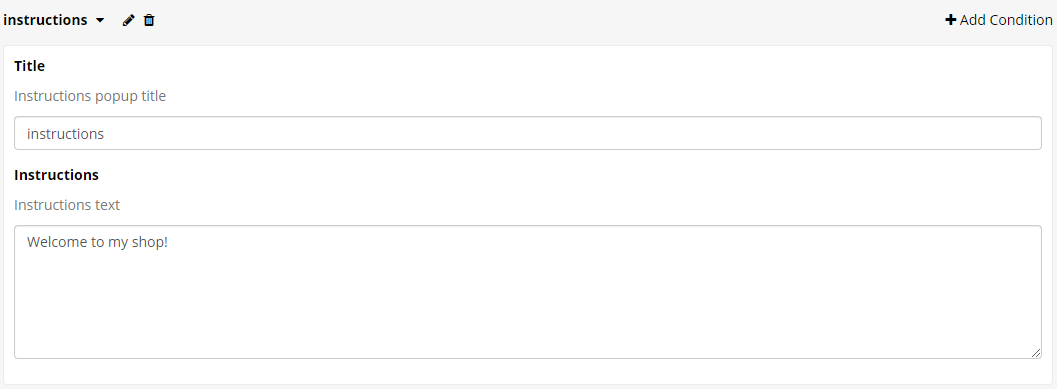The image depicts a user interface component designed for entering a title and instructions. At the top is a section labeled "Instructions" with a drop-down box. On the right, there is an edit button followed by a trash can icon at the far right. To add a new condition, a plus sign is also placed in this section. This entire segment is distinguished by a gray bar.

Below the gray bar, a white box stretches from the left to the right edge of the interface, starting flush with the instruction title. Inside this white box, the word "Title" appears in black text. Further below, "Instructions" is written in bold, followed by two text areas for entering different sets of instructions. 

The first text area labeled "Title" appears in gray, indicating a pop-up title field. Adjacent to it is a text box labeled "Instructions," also encased in a white box stretching the full width, designed for longer input. 

The second set of fields is similarly structured. It starts with a bold "Instruction" label, below which there is gray text that says, "Instructions text." Beneath this, in a large white text box, the phrase "Welcome my shop" is displayed, with "Welcome" capitalized and "shop" emphasized as though shouted. This text area is spacious, allowing for extensive input. 

Overall, the visual layout features a light gray bar at the top followed by white text boxes, each clearly labeled and designed for user-friendly input of titles and instructions.